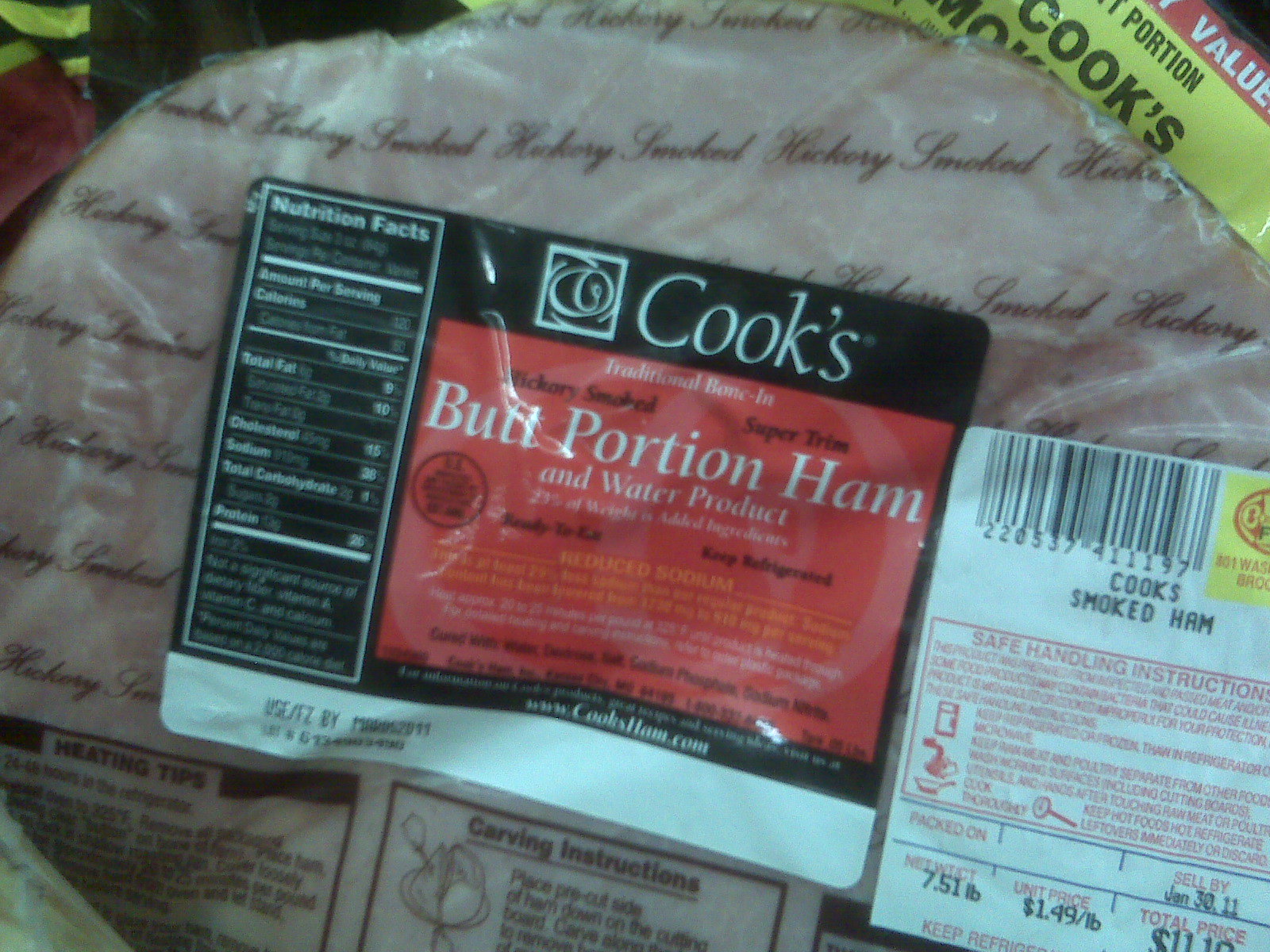The photograph is a close-up image of a plastic-wrapped piece of ham, specifically zooming in on the nutrition facts and various labels. The ham is encased in clear plastic, adorned with cursive text reading "Smoked Hickory" in black font. A prominent black label occupies a significant portion of the packaging. At the top of this black label, the word "Cooks" is displayed in white font. Below, within a red square on the same black label, the text "Butt Portion Ham and Water Product" is clearly visible. The fine print surrounding this text is too small to decipher. 

To the left of the central label, the nutrition facts are presented, also in white font against the black background. At the bottom of the black label, there is a white bar indicating the expiration date, though the text is too tiny to read. In the lower right corner of the packaging, a white price tag shows the cost of the product as $11.10.